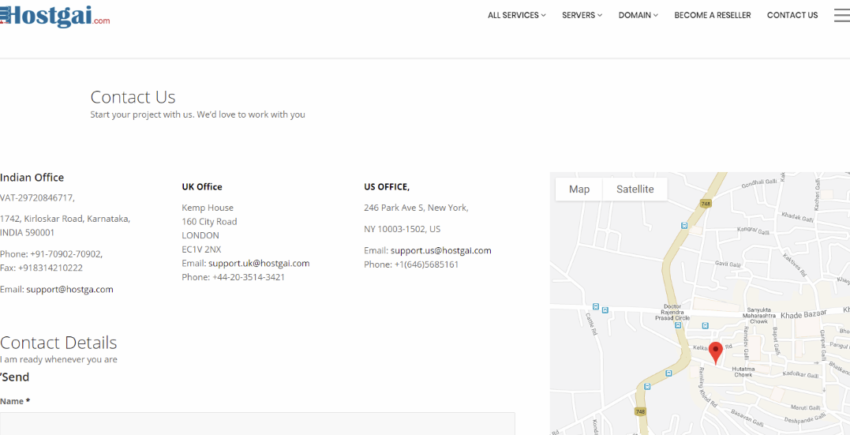In the upper left corner of the image, blue text spells out "h-o-s-t-g-a-i.com." To the right, a series of links are displayed: "All Services," "Servers," "Domain," "Become a Reseller," and "Contact Us." Below these links, a gray text section invites viewers to "Start your project with us. We'd love to work with you," followed by contact details for different office locations.

The Indian office information includes a phone number and fax number. The UK office is located at 160 City Road, London, with an email address provided. The US office is at 246 Park Avenue, New York, again with an email address and phone number listed.

To the right side of the image, a map section is visible, offering both Map View and Satellite View options. The map displays a long, curving yellow line representing a road, dotted with small blue squares indicating different areas along the road. A prominent red dot on the map marks one of the office locations, which appears to be based in the United States. Additionally, contact details corresponding to these locations are displayed on the left side of the map.